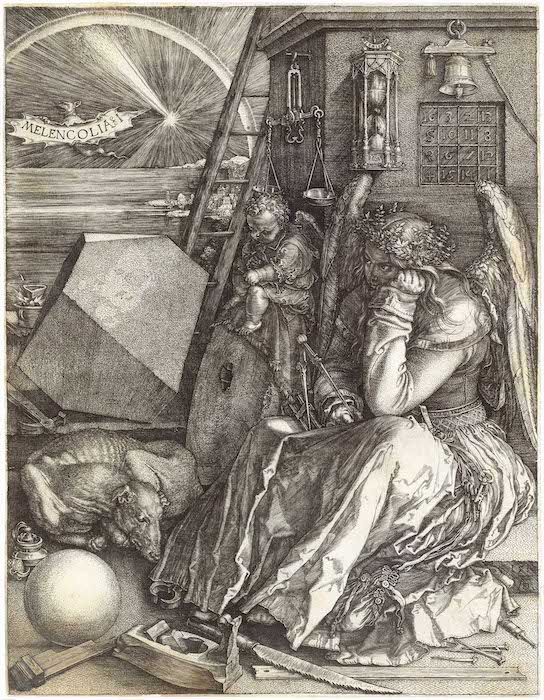This vintage-style black and white pencil drawing captures a detailed scene brimming with symbolism and intricate elements. At the forefront, there is a large adult angel sitting pensively on a porch, her head resting on one hand, dressed in a flowing robe and adorned with majestic wings. Beside her is a smaller, cherubic child angel, engaged in some activity with its hands. In the surrounding environment, there are numerous fascinating details: a half-starved dog stands in front of the angels, while various objects like a sphere, wooden implements, and possibly sculpting tools lie scattered about, suggesting an unfinished task or artistic endeavor. To the right side, a formidable tower with a ladder leading up its side glances into the scene, with a bell and an hourglass positioned in the foreground. The background reveals a port, hinting at a broader world beyond this moment. Above, in the top left corner, a luminous sky—presumably illuminated by the sun or moon—casts a radiant light over the scene, while a banner reading "MELENCOLIA I" underscores the theme of melancholy. The entire composition is rendered with meticulous detail, utilizing crosshatching and stippling techniques to create depth and texture, and it spans edge to edge without any framing.